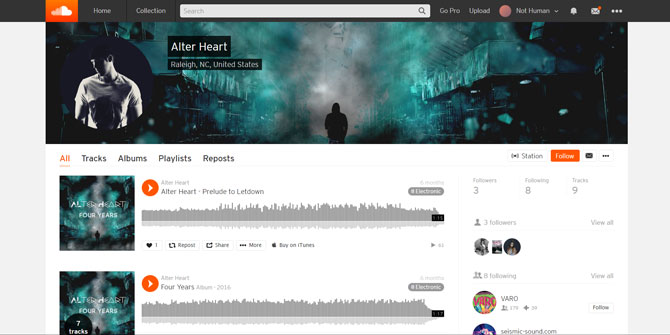This image depicts a detailed screenshot of a music app or playlist interface. At the very top, there is a black bar, beneath which, on the left, is an orange box featuring a white cloud icon. Adjacent to it, the words "Home" and "Collections" are displayed in white text. The center showcases a large white search bar adorned with a magnifying glass icon and the word "Search." To the right of this bar is "GoPro Upload" in text alongside a red circle. Further to the right is an indication that says "Not Human" with an arrow, followed by a notification icon and an envelope marked with an orange dot, signifying new mail. Three dots line up next to the envelope icon for additional settings.

Below this navigation area, there's an image titled "After Heart" with Raleigh, North Carolina, United States noted beneath it. The image is circular and features a man in a white T-shirt, possibly with a black design, looking to the right. The background is predominantly black, portraying a dilapidated street scene at night, potentially reminiscent of a post-apocalyptic scenario. The buildings appear in disrepair, and a silhouetted figure is walking down the middle of the street under grayish-black hues with light gray shadows.

Beneath this image, various sections are listed in orange and black text: "Tracks," "Albums," "Playlists," and "Reposts." To the right is a station icon, reminiscent of a radio station, within an orange box, followed by a black chat icon and three dots for more options.

On the left of the interface, there are additional images and sections echoing the main display. The first picture reiterates "After Heart" with a note of "four years" and to the left another with the same phrase. Inside the second image, a black circle notes "seven tracks." Adjacent to the first image is an orange circle with an arrow, and the text "After Heart Preload to Let Down" is displayed alongside a grey-lined graph, typically representing sound waves.

Further details under this section show "Followers: 3," "Following: 8," and "Tracks: 9," with a small icon of a person and an option to "View All." This section includes profile images, though some are too indistinct to discern.

Continuing, the left sidebar mirrors the earlier elements. An orange circle says "four years" and "Albums: 2016" under another "After Heart" mention. The lines graph appears again in gray. The text includes an obscured gray text box and additional following stats. Profile picture circles follow; one's labeled "Borrow," and another cuts off but hints at a blue image with a mention of csound.com.

Lastly, at the bottom of each of these sections, a small black box presents timestamps, one approximated as "9:14" and another as "9:17," though they are somewhat blurry.